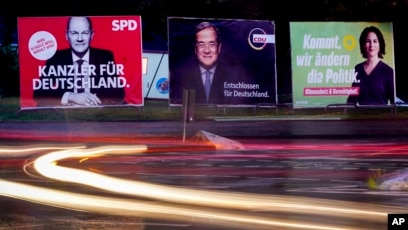In a dynamic, outdoor setting captured photographically, this image showcases a vibrant racetrack at night, with cars speeding around the track, their yellow and red lights blurring into streaks due to their rapid movement. Above the racetrack, three billboards stand prominently against the dark sky, each displaying different political advertisements in German. The leftmost billboard features a balding white man in a black and white suit with the words "Kanzler für Deutschland SPD." The middle billboard displays another man, possibly Asian, wearing a blue suit and tie, with text partially spelling out "ENTICHLÖWEN für Deutschland" alongside the letters "C-D-E-U." The rightmost billboard highlights a woman with the inscription "KOMMT, wo ANDIENDIE Politik." At the bottom right of the image, a small black rectangle with white "AP" letters suggests this might be a snapshot from a newscast, further supported by the overall scene and the German text indicating political campaign messages. Bright curved light trails in the foreground add to the energetic ambiance of the scene.